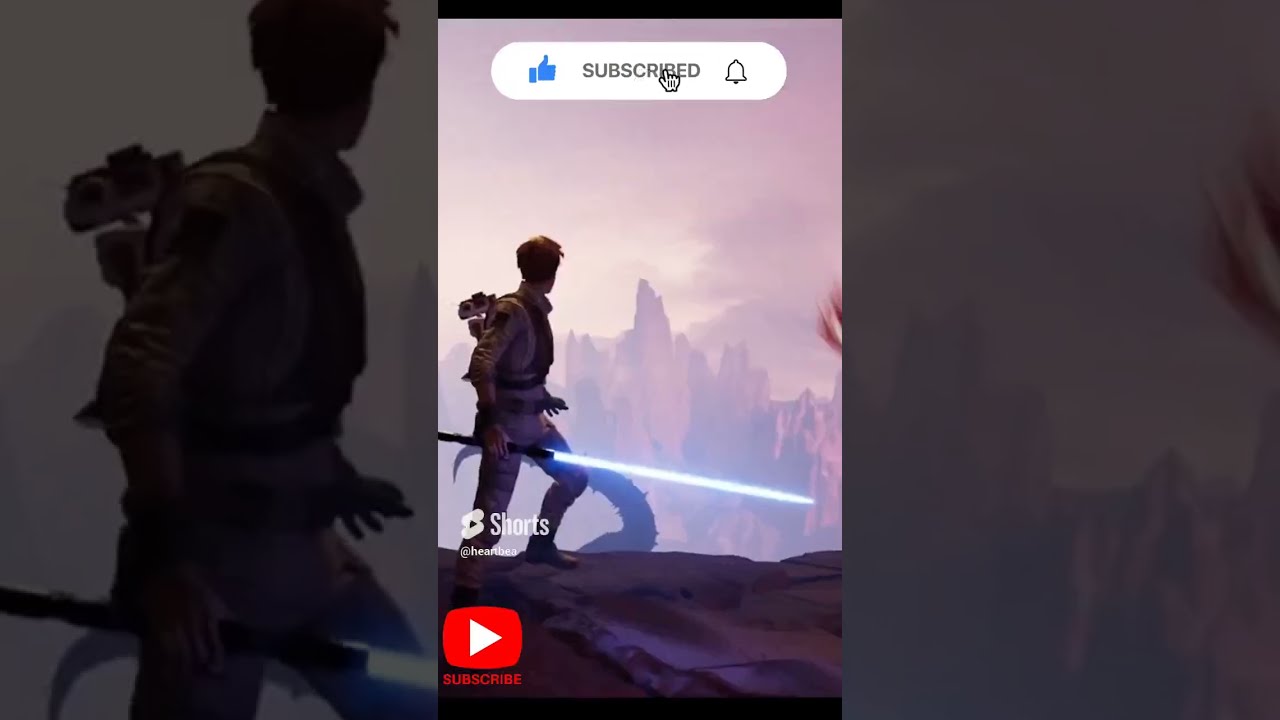The image is a screenshot from a YouTube Shorts video displaying a Star Wars Jedi character. The vertical cell phone picture shows the main image centered, with the same picture zoomed in on both the left and right sides. The Jedi, standing on a rocky surface, is holding a blue lightsaber in his right hand and has a robot's head peeking out of a backpack. He faces left, gazing into the distance, where a rocky cliff and an overcast, brown sky form the backdrop. A tentacle-like monster's arm with a sharp point protrudes from the ground behind him. The top of the image features a blue thumbs-up icon with "subscribe" text, while the lower-left corner displays a YouTube Shorts logo and an unreadable YouTuber's name above a red subscribe button.